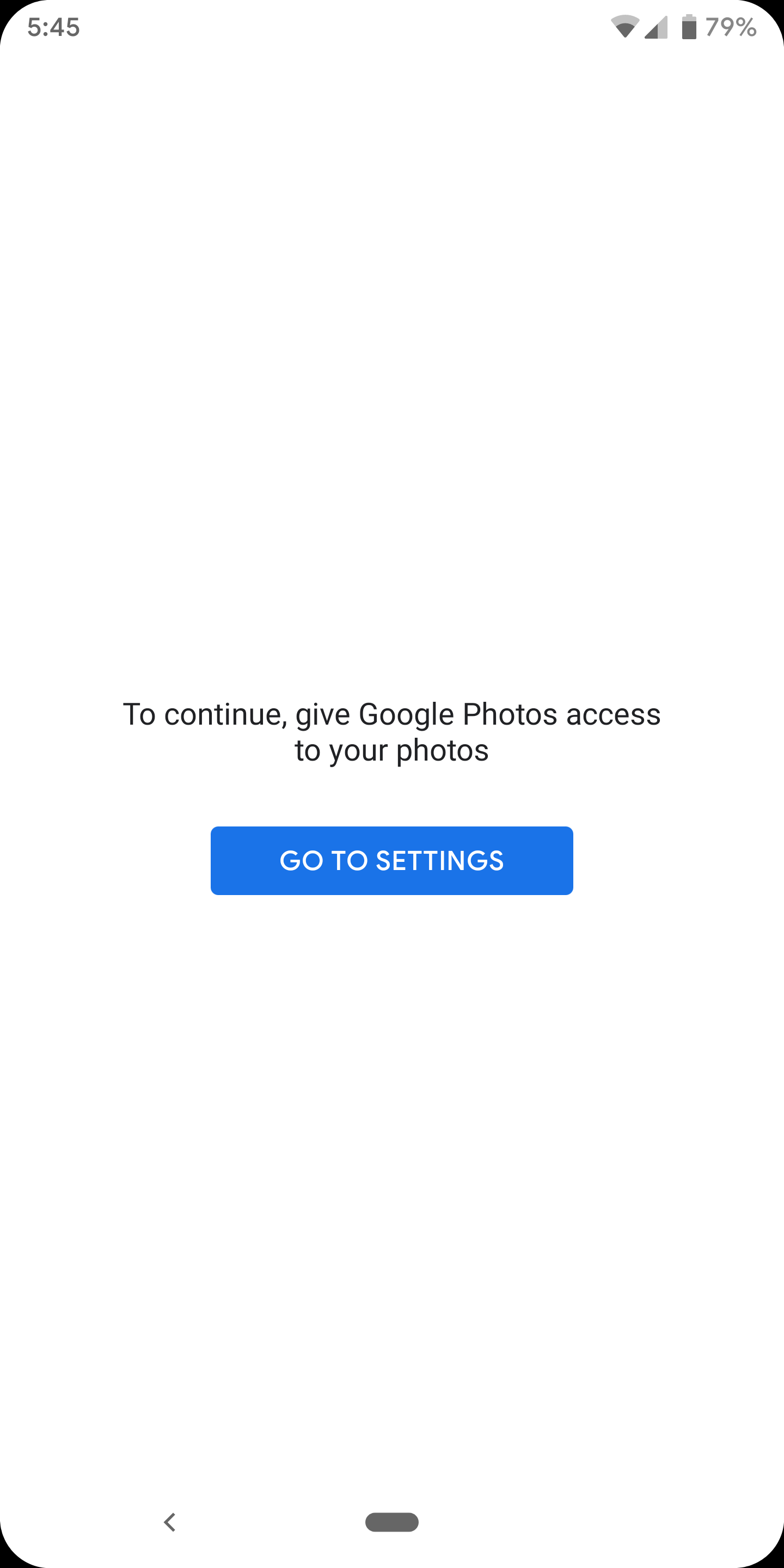A screenshot taken from a phone, showcasing a minimalistic and straightforward interface. The overall screen is predominantly white, with black triangles in each corner. 

- **Top Left Corner:** Displays the time "5:45". 
- **Top Right Corner:** Icons for Wi-Fi signal, network signal, and battery status, with the battery indicated at "79%".
  
At the bottom of the screen, a gray navigation bar is visible, featuring a central home button and a back arrow button to the left.

In the center of the screen, a message in black text reads: "To continue, give Google Photos access to your photos." Below this message, a blue button with white uppercase text prompts the user to "GO TO SETTINGS".

The image is devoid of any additional visuals or text, creating a very plain and utilitarian appearance focused solely on the prompt and navigation elements mentioned.